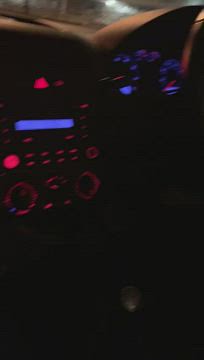The photograph captures the interior of a car at night, focusing on the dashboard. The scene is dimly lit, suggesting it's taken in low-light conditions with street lights faintly reflecting off the top of the dashboard. Dominating the center of the image is the center console. Near the top, an orange-reddish triangle is prominent, positioned just above a blue rectangle likely representing the stereo system, surrounded by various buttons and lights. These buttons and lights are illuminated in a warm orange hue. Beneath these controls are three circular dials glowing red, presumably for climate control. Lower still, the gear lever is barely visible in the shadows. To the right, the gauge cluster comes into view, its speedometer and odometer bathed in the same blue light as the stereo in the center console. The steering wheel's outline is also faintly visible, framing the driver's viewpoint.